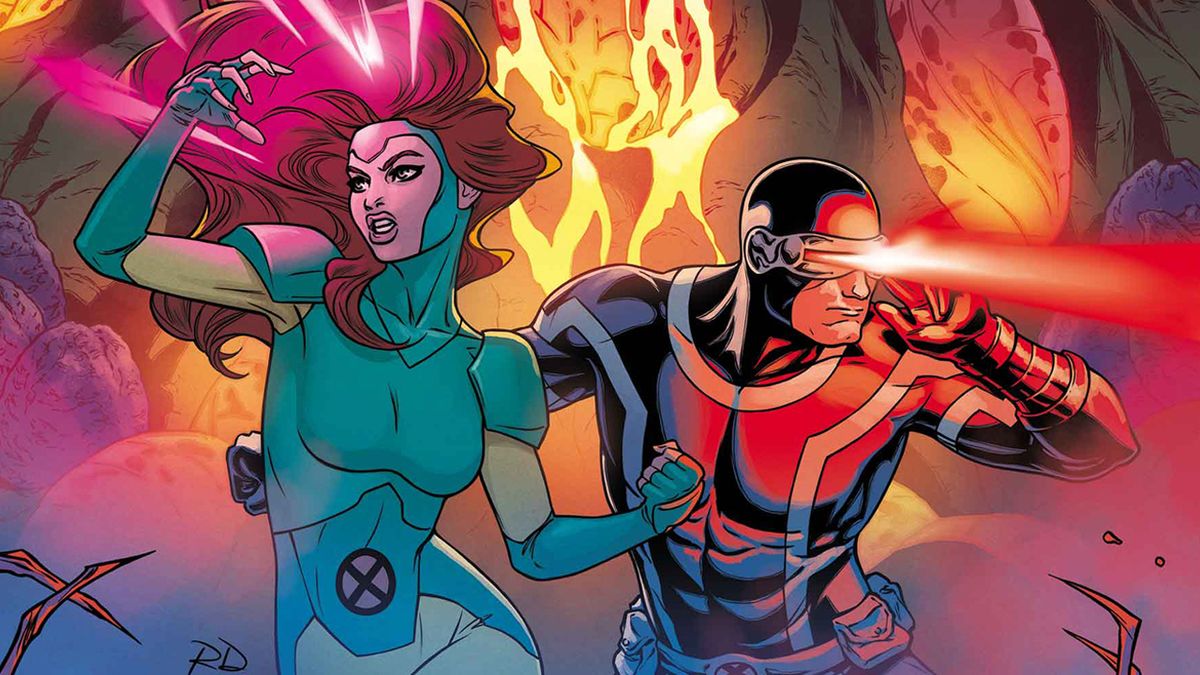The image, reminiscent of a Marvel comic book illustration by Russell Dauterman, portrays two striking characters set against a vibrant and chaotic background. On the left, a female character with voluminous, flowing dark red hair, partly covered by a green outfit that ascends to form a half-helmet around her head, exposing only her ears. Her right hand is clenched into a fist and positioned close to her head, while her left hand is extended with fingers splayed, as if blocking or casting something. This woman wears a skin-tight suit, predominantly green with teal shoulder pads and gloves, and a light cream section below her waist. A black circle with a red X, indicative of the X-Men logo, adorns her stomach area. Her fierce expression, complete with a gritted mouth, is accentuated by purple lightning bolts radiating from her hair.

To the right is a male character in a metallic, skin-tight suit reflecting the reds, yellows, and oranges of their fiery background with dark blue and black shadows. He dons a metal helmet with a visor over his eyes, from which a piercing yellow light beams out, bleeding into a bright red. His visible facial features include the chin, mouth, and nose, as he maintains a stoic demeanor. Around his waist is a fanny pack, adding practicality to his sleek, muscular appearance.

The backdrop is a tapestry of chaos and color, featuring a central eruption of fire with a landscape painted in magenta, purple, and orange hues. Lava flows from a rocky formation on the right side of the image, while on the left, purple bushes silhouette against the colorful maelstrom.